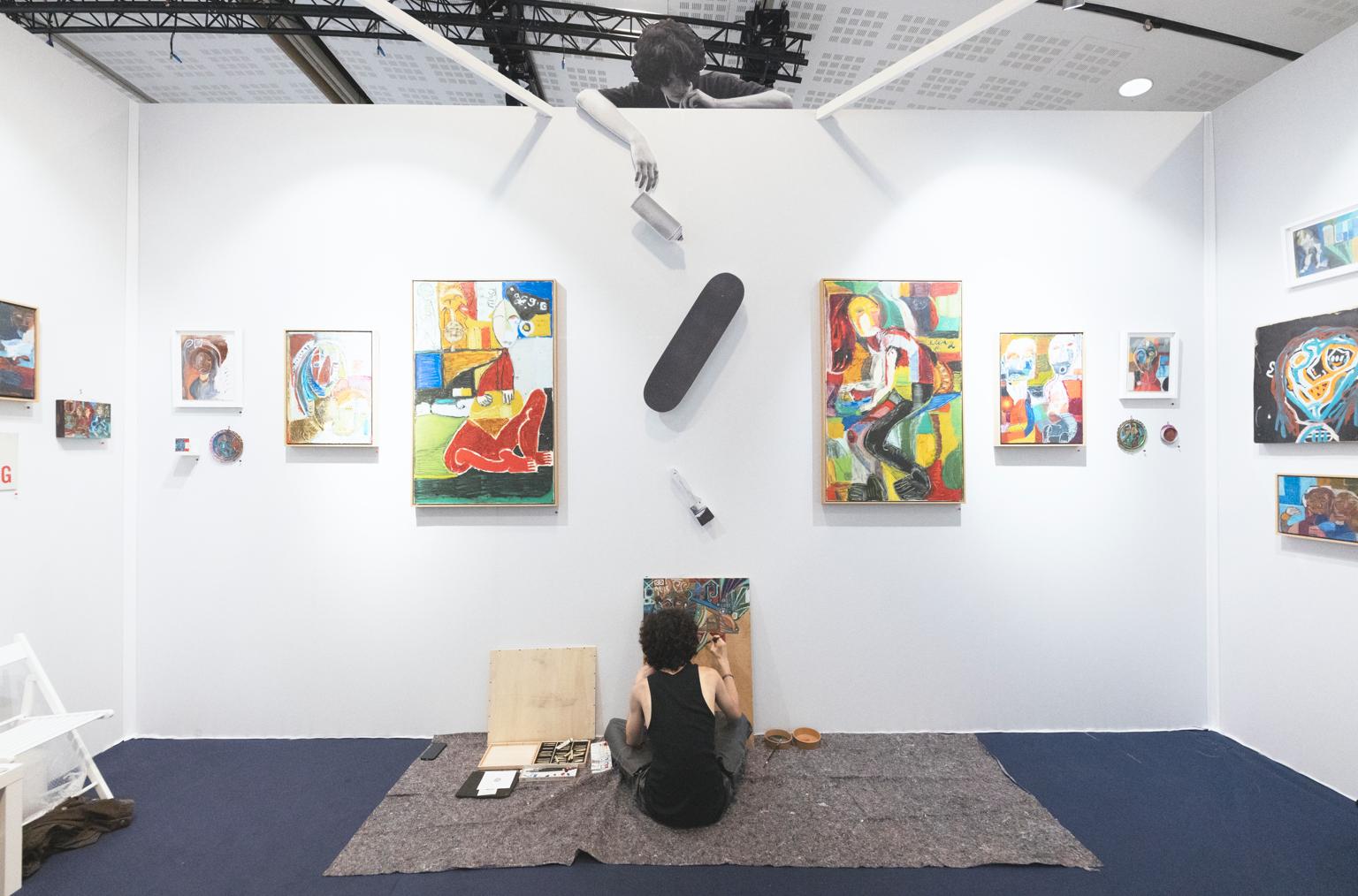In a staged, full-color indoor photograph illuminated by artificial light, the scene is set in what appears to be an art studio. The image, horizontally rectangular in format, captures a moment where two individuals are engaged in an artistic activity. The foreground showcases a man seated on a gray rug over a blue floor, absorbed in painting on a brown canvas. He has dark curly hair, wears a black tank top and gray or tan pants, and is surrounded by a box of pins and colors placed on the floor to his left.

The studio's walls, painted white, form a U-shape surrounding the painter, adorned with around ten abstract paintings, with the largest canvases prominently hanging directly above him. In the background, another figure, seemingly dressed in black and appearing almost monochromatic in contrast to the rest of the image, leans over from the top of the wall, holding what looks like a can of spray paint.

The ceiling is visible, featuring black piping or scaffolding that runs from the top left into the middle of the frame. The unusual inclusion of a small, black object resembling a skateboard, yet too small to function as one, is positioned dead center, adding an intriguing element to the staged composition. This carefully arranged scene highlights the dynamics within an art studio, combining the act of creation with a touch of the surreal.